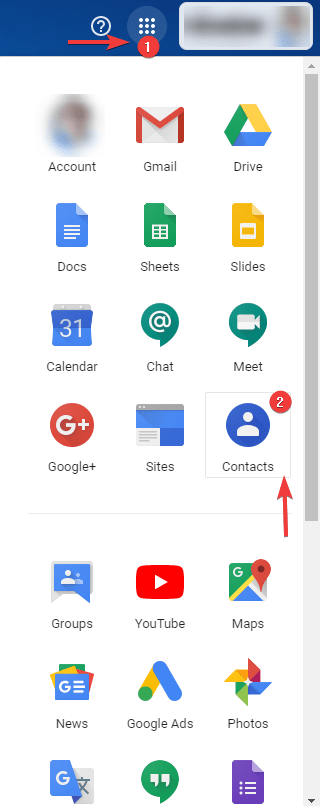A detailed caption for the image could be:

"This image features a composite screenshot of a smartphone's home screen, displaying a variety of app icons organized in a grid layout. The screenshot appears to be stitched together, showing two different sections of the home screen, separated by a faint horizontal line. At the very top of the image, a blue menu bar can be seen, typically indicative of the main menu interface.

The background of the screen is white, providing a clean canvas for the colored app icons. Each row contains three icons, making it easy to distinguish individual apps. The first set of rows showcases popular Google apps: Gmail, Google Drive, Docs (blue icon), Sheets (green icon), Slides (yellow icon), Calendar (blue icon with the number '31'), Google Chat, Google Meet, Google Search, Google Sites, and Contacts.

Below the horizontal separator, the next set of rows includes additional Google services and other commonly used apps: Groups, YouTube, Maps, News, Google Ads, and Photos. The image cuts off before displaying additional icons, suggesting there are more apps present beyond what is shown.

Overall, the structure and arrangement of the app icons make it visually similar to a typical user's organized but comprehensive app library on a smartphone device."